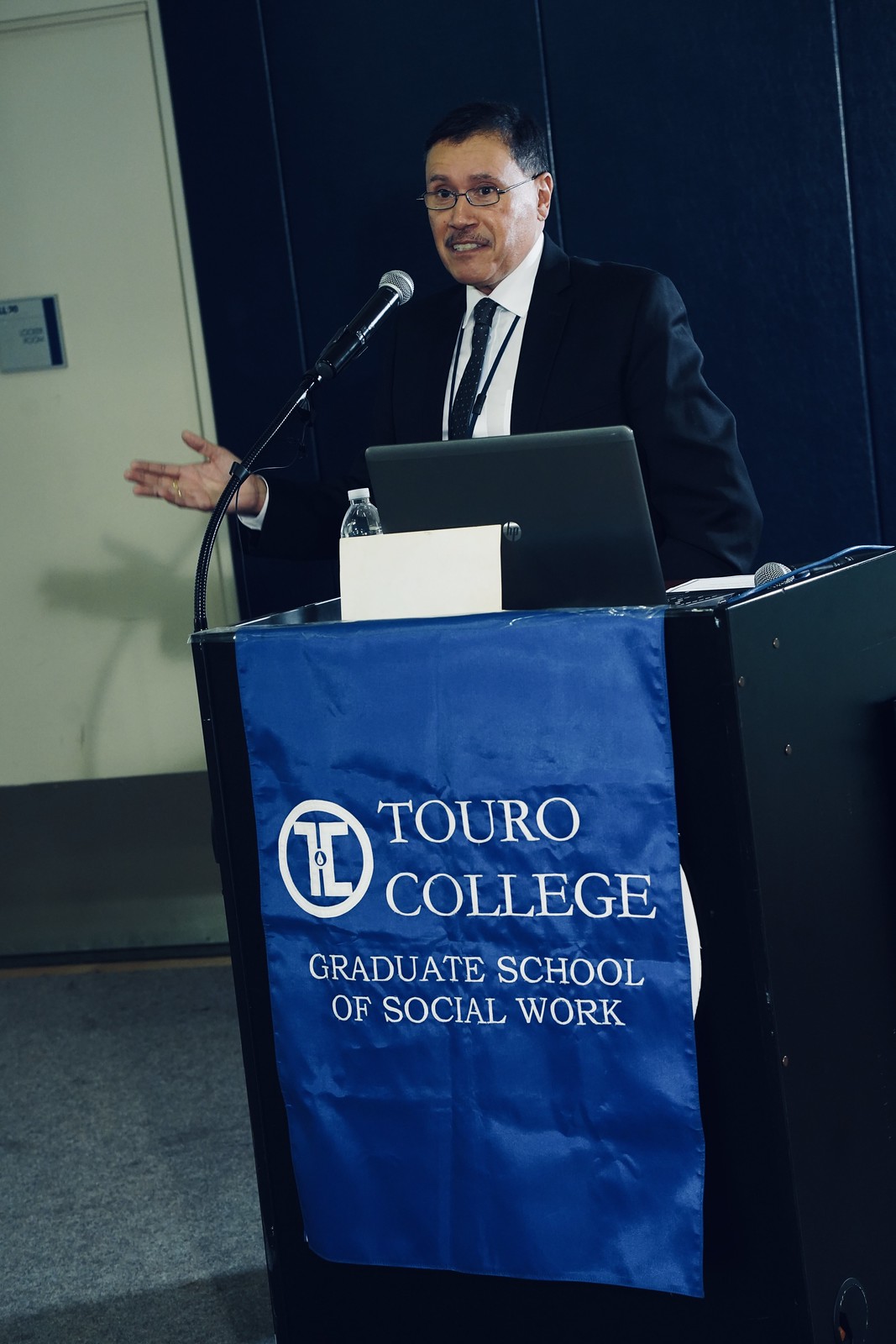In this detailed color photograph, a man in his early 60s is speaking at a podium adorned with a blue satin banner. The banner reads "Touro College Graduate School of Social Work" in white text, complete with a circular logo featuring the letters "TC." The man is dressed formally in a black suit with a white collared shirt and a dark tie, and he wears black-framed glasses with clear lenses. He has dark hair, a mustache, and a placard around his neck. He is gesturing with his right hand while addressing the audience through a black microphone curved towards his face. On top of the black podium, there is an open black laptop and a small water bottle. The background features a white wall on the left and a darker area on the right, capturing a moment of engaged oration reflective of photographic realism.